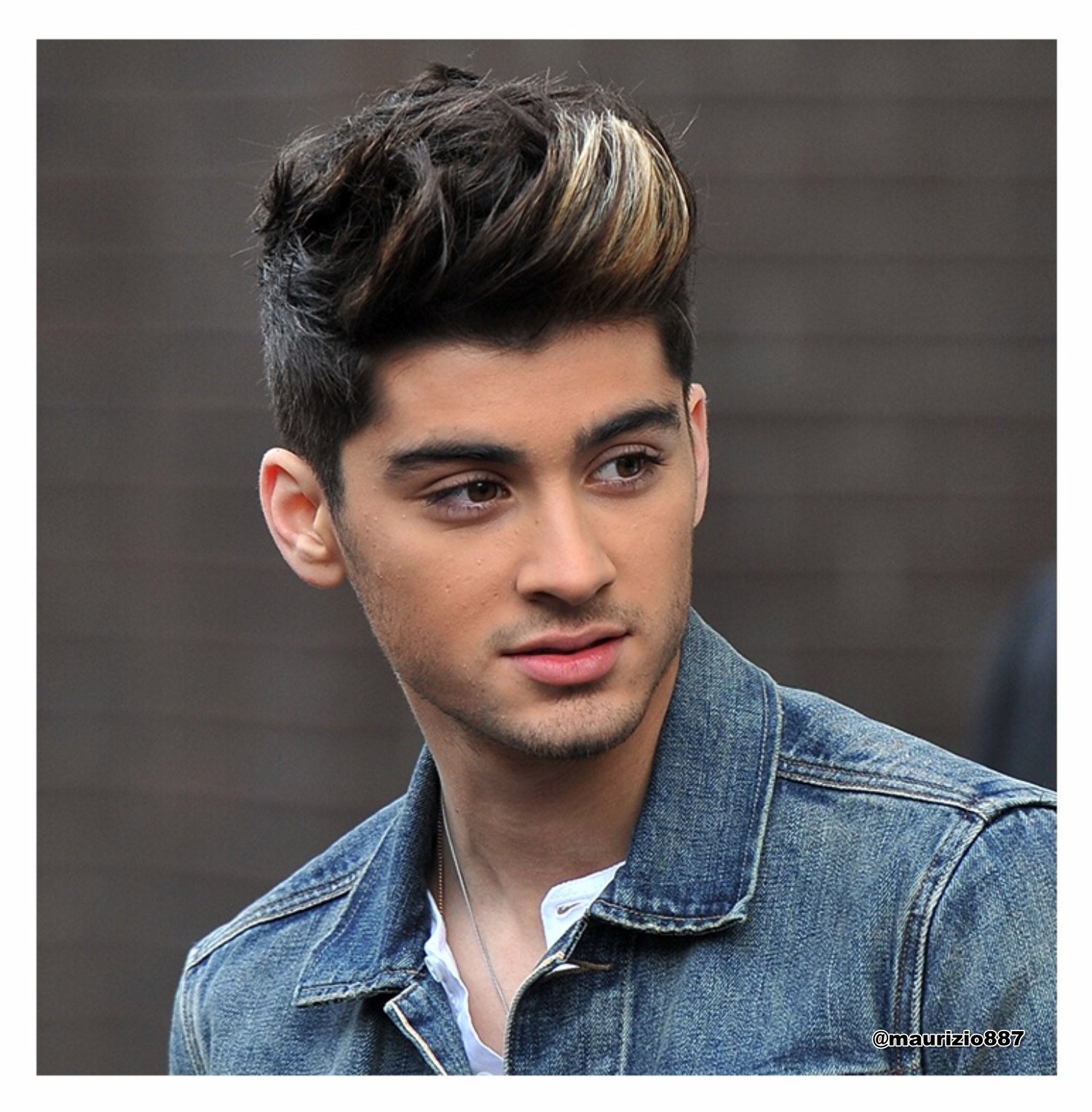This square photograph features a young man from the shoulders up, with his right shoulder cropped out on the right side and his left shoulder extending to the bottom edge of the image. He sports a serious expression, looking slightly downward and to his right. His light brown skin contrasts with his dark brown hair, which has blonde streaks and is styled upwards with gel. His dark black eyebrows stand out against his face, which shows faint signs of a mustache and beard. The man is dressed in a white shirt underneath a denim jacket, and he is adorned with two necklaces—a silver one in clear view and a partially hidden gold one. The gray background behind him is decorated with horizontal stripes, adding subtle texture to the image. In the bottom right corner, the photo is tagged with "@Maurizio887" in black font.